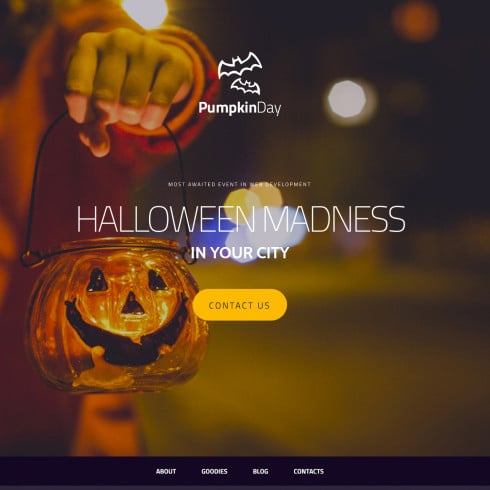The image on the page appears to be an advertisement or a section of a website, focused primarily on a visually captivating background rather than text. The background features a person holding a glass jack-o'-lantern lamp, artistically designed with the traditional facial features of a jack-o'-lantern. The person’s head is not visible, only a partial view of their body and a hand clasping the lamp are shown. The lamp is held up against a backdrop of blurred street lights, giving a mysterious and atmospheric touch to the scene.

In the foreground, several textual elements are displayed. At the top, in white text, are the words "Pumpkin Day" accompanied by two bat icons on either side. Below this, there's a caption that reads, "The most awaited event in WGN development" followed by "Halloween madness in your city." Toward the lower part of the page, a prominent yellow "Contact Us" button is visible. Finally, covering the bottom section is a black bar containing the navigation options: "About," "Goodies," "Blog," and "Contacts," all depicted in white text.

Overall, the layout visually prioritizes the festive and eerie mood evoked by the glowing jack-o'-lantern lamp, enhanced by the blurred urban background.